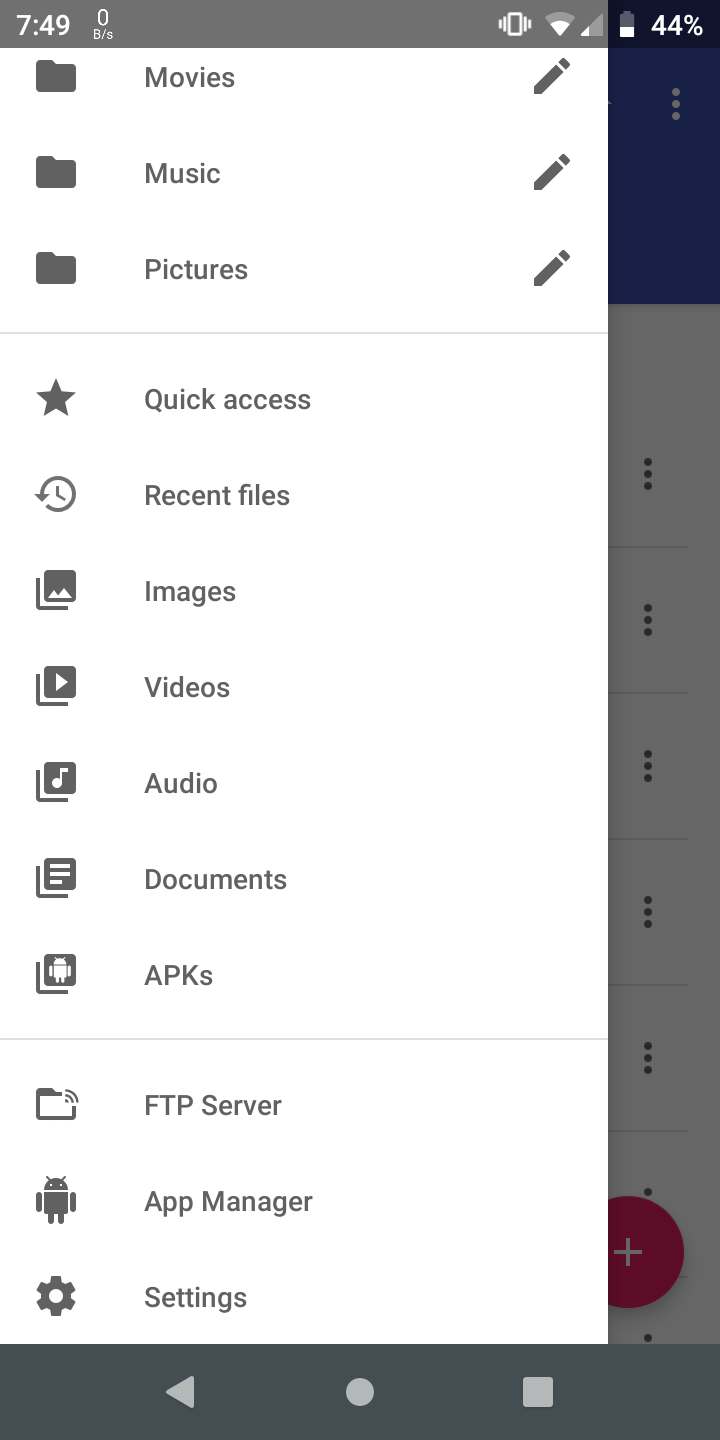**Screenshot of File Management Interface**

The screenshot displays a file management interface, delineated into various sections for easy navigation. 

At the top, there is a heading that categorizes the files into "Movies," "Music," and "Pictures," with each section marked by their respective icons. The text is colored in gray on a pristine white background. Beneath the headings, there's a set of icons resembling pens, likely indicating editable options or file attributes.

A thin gray line separates this section from the "Quick Access" area, which features noteworthy icons and indicators:

1. A star icon labeled "Quick Access."
2. A clock icon depicting a reverse-chronological timeline with the label "Recent Files."

In the middle of the interface, file type categories are represented by specific icons:

- A photo icon for "Pictures, Images, Videos."
- A musical note for "Audio."
- Bar graph icon for "Documents."
- A small robot for "APK files."

A gray line further segments the categories from the additional options below:

- An icon labeled "FTP Server."
- Another robot icon marked "App Manager."
- A gear icon denoting "Settings."

Towards the bottom, the interface also displays standard Android navigation buttons - a square, a circle, and a triangle.

Additionally, a battery indicator displays 44% remaining battery life. To the lower right, a red circular button with a white plus sign sits, likely for adding new files or folders.

Finally, the interface concludes with eight rows, each with seven vertical dots, possibly indicating more detailed settings or further navigation options.